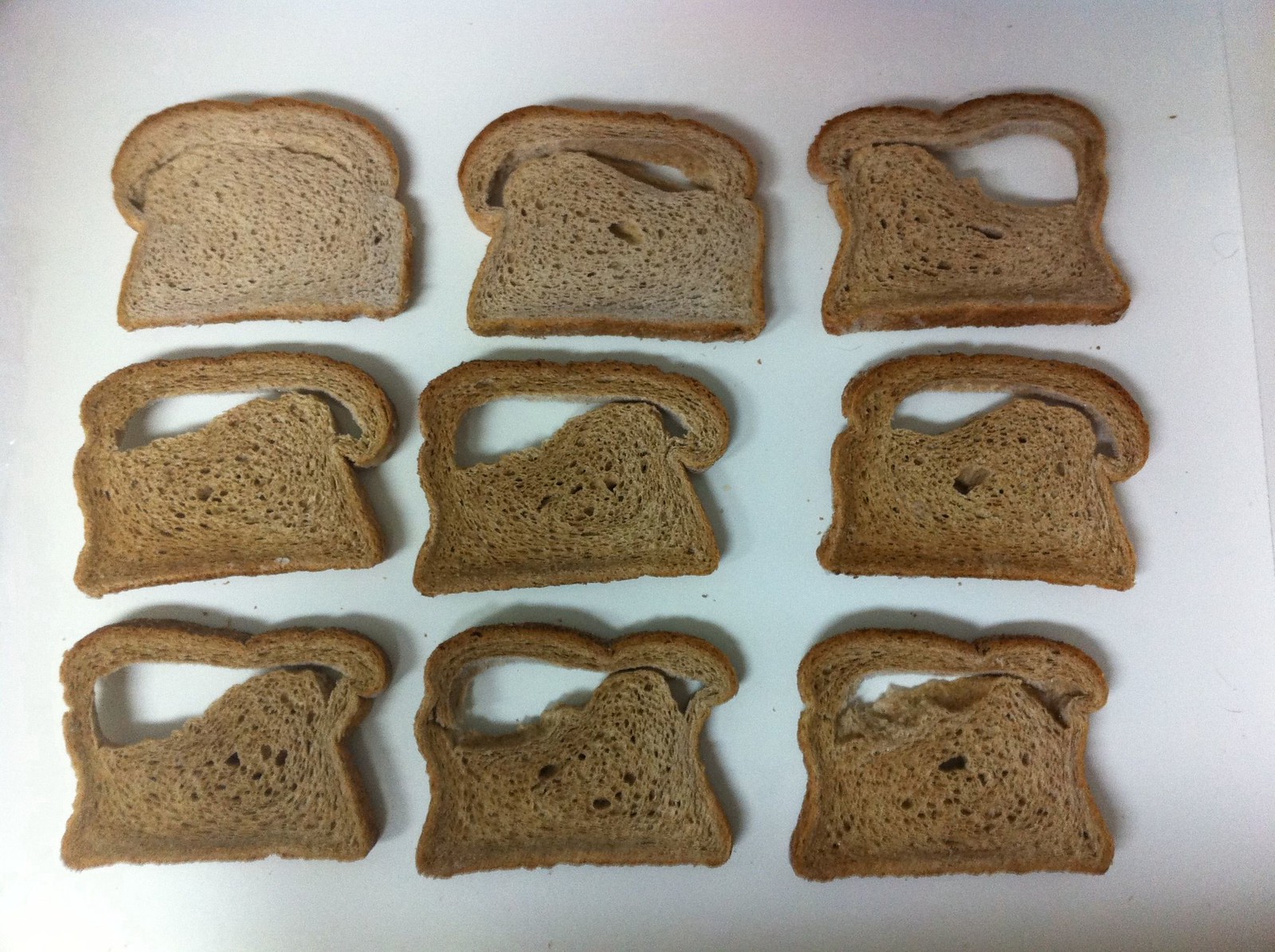The image displays a detailed, color photograph in a landscape orientation featuring nine slices of wholemeal brown bread arranged in a three-by-three grid pattern against a white background. Not perfectly aligned, the slices are spaced out, all oriented with the rounded tops, or double bumps, facing upward. The slices exhibit various irregularities due to air bubbles in the baking process, resulting in significant holes, predominantly near the crust area. Among them, the slice in the upper left is the lightest in color and appears intact, contrasting with the others that exhibit noticeable gaps and slits. The slice in the center of the top row has a horizontal slit, while the one in the upper right shows a large hole at the top right. The middle row slices vary slightly in shape, each expanding more on the left and tapering on the right. On the bottom row, the left and center slices have large holes on the left side, whereas the right slice shows a smaller hole on the left. The white background changes in shade from lighter at the top to darker toward the bottom. The photograph also captures the texture and slight shadows of the bread, suggesting a light source from the left bottom corner, creating longer shadows on the bottom row and shorter ones on the top row, adding depth to the composition.